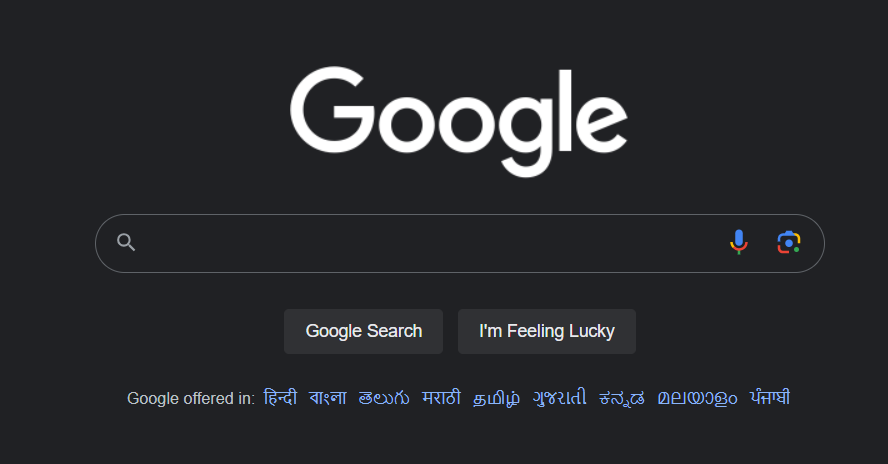In this image, there is a horizontally oriented rectangle set against a completely black background. The layout appears to mimic a Google search page. The prominent "Google" logo, featuring a capital 'G' followed by lowercase letters, is displayed in white font at the top. Below the logo, a search bar is outlined in gray. To the left side of the search bar is a gray magnifying glass icon, signifying the standard search function. On the right side of the search bar, there is a blue microphone with yellow, green, and red accents, indicating voice search capability. Additionally, a multicolored camera icon—also in blue, yellow, green, and red—signifies the option to search using images. Below the search bar, there are two buttons: one labeled "Google Search" and another labeled "I'm Feeling Lucky."